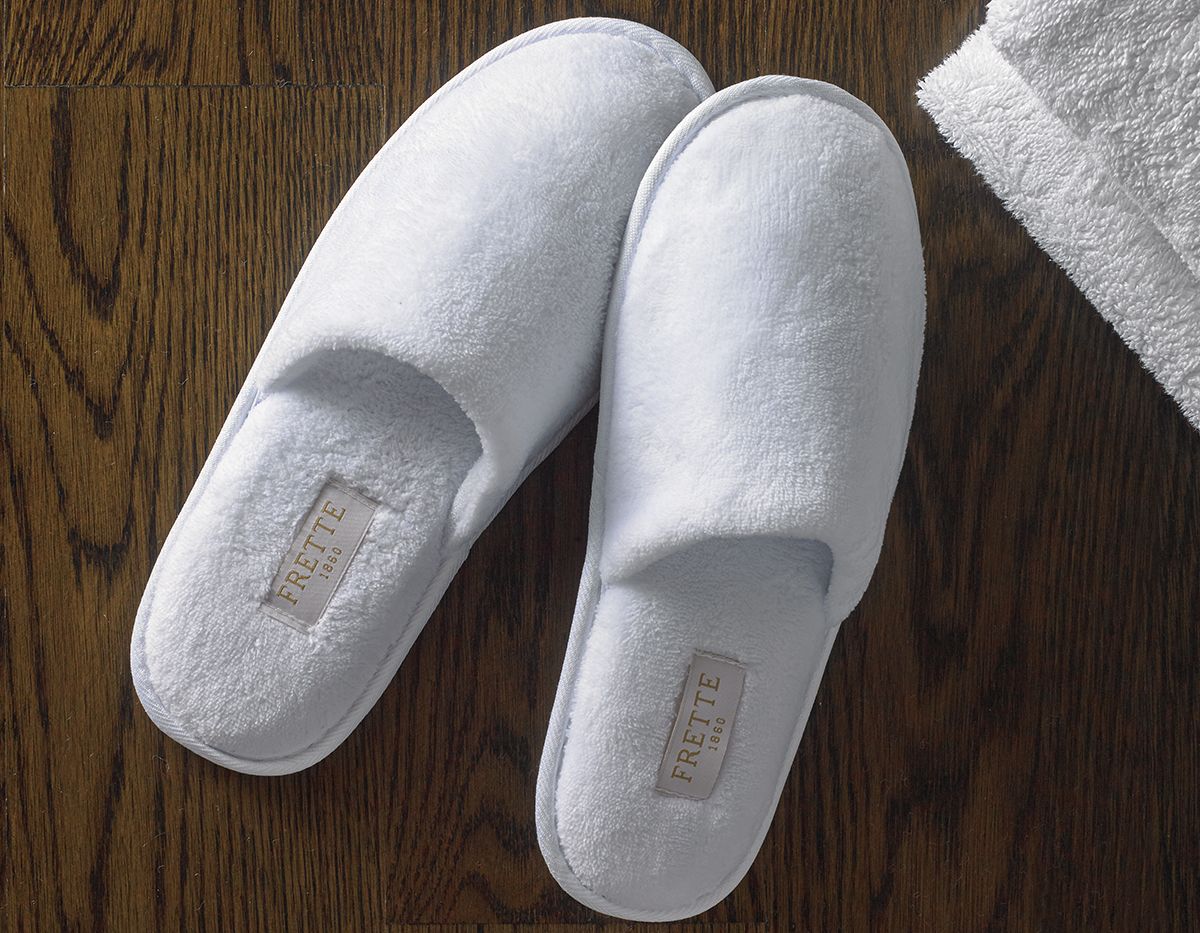The image depicts a pair of pristine white slippers with a cozy, towel-like texture, positioned slightly overlapping on a polished wooden floor. The right slipper extends over the toes of the left slipper. A label is affixed to the rear of each slipper, reading "FRETTE" in bold, capitalized, bronze-colored letters, with the year "1860" written underneath. In the upper right corner of the frame, there is a visible portion of neatly folded white towels or possibly a bathrobe. The wooden floor beneath the slippers showcases a well-maintained, medium brown, slatted pattern, reflecting a clean and polished appearance. The overall ambiance hints at a luxurious setting, perhaps akin to what one might find in a high-end hotel room.